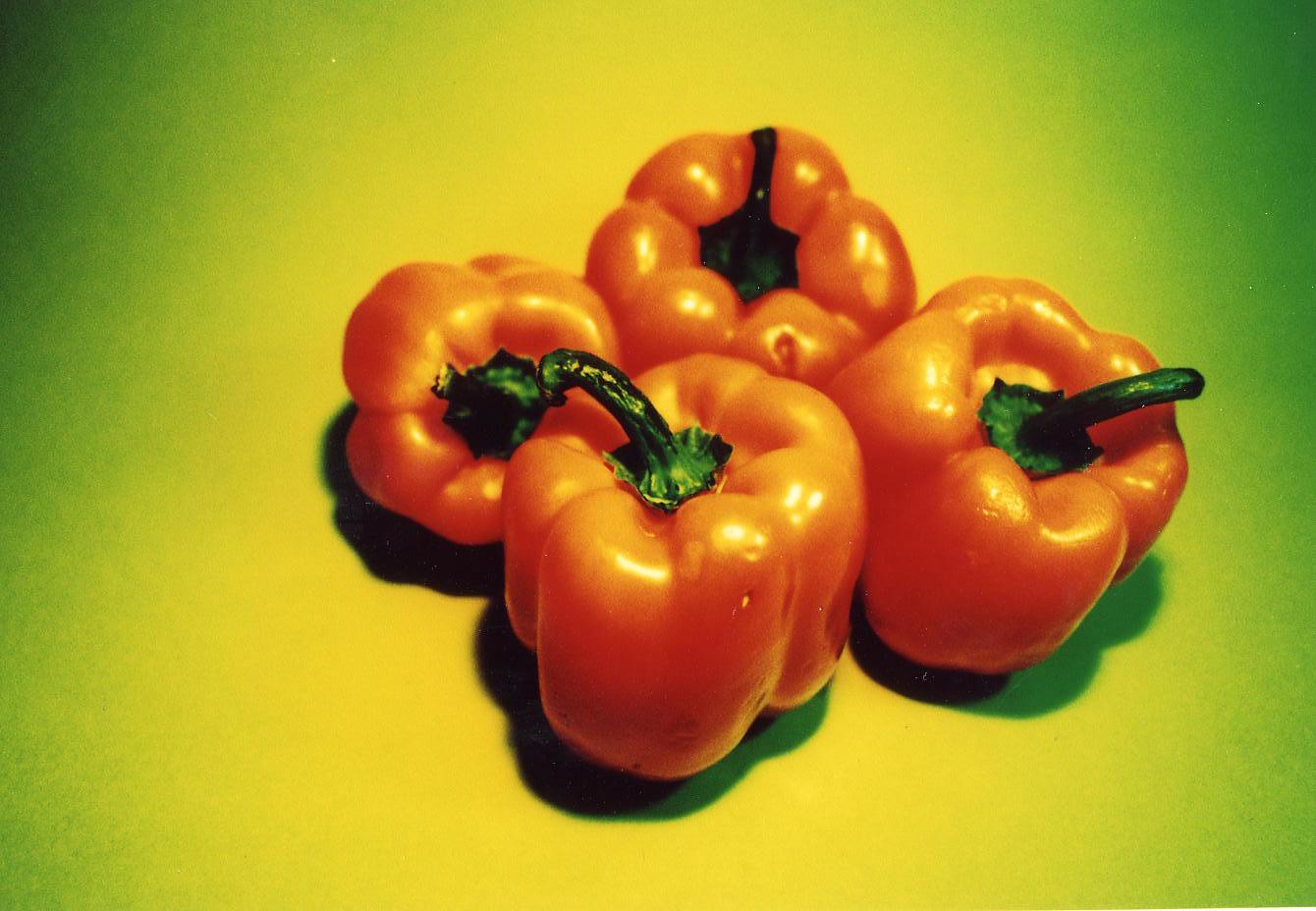In this artistic image, which could be mistaken for a computer-generated graphic or a painting, we observe a striking composition of four peppers set against a vivid background. The backdrop transitions from green at the edges to yellow towards the center, creating a gradient effect that emphasizes the focal point. Positioned slightly to the right of the center, the four oranges peppers form a loose plus sign. Three of the peppers stand upright, while the fourth, in the top left, leans on its side towards the first pepper. These peppers are notably glossy, exhibiting a shiny surface that casts distinct shadows, particularly from the front two and the slanted one. Each pepper features a green stem, adding contrast. Despite their polished appearance, there are minor imperfections on the peppers, indicating a photorealistic quality. The interplay of light and shadow reinforces the depth and realism of the scene, making the peppers appear almost tangible.